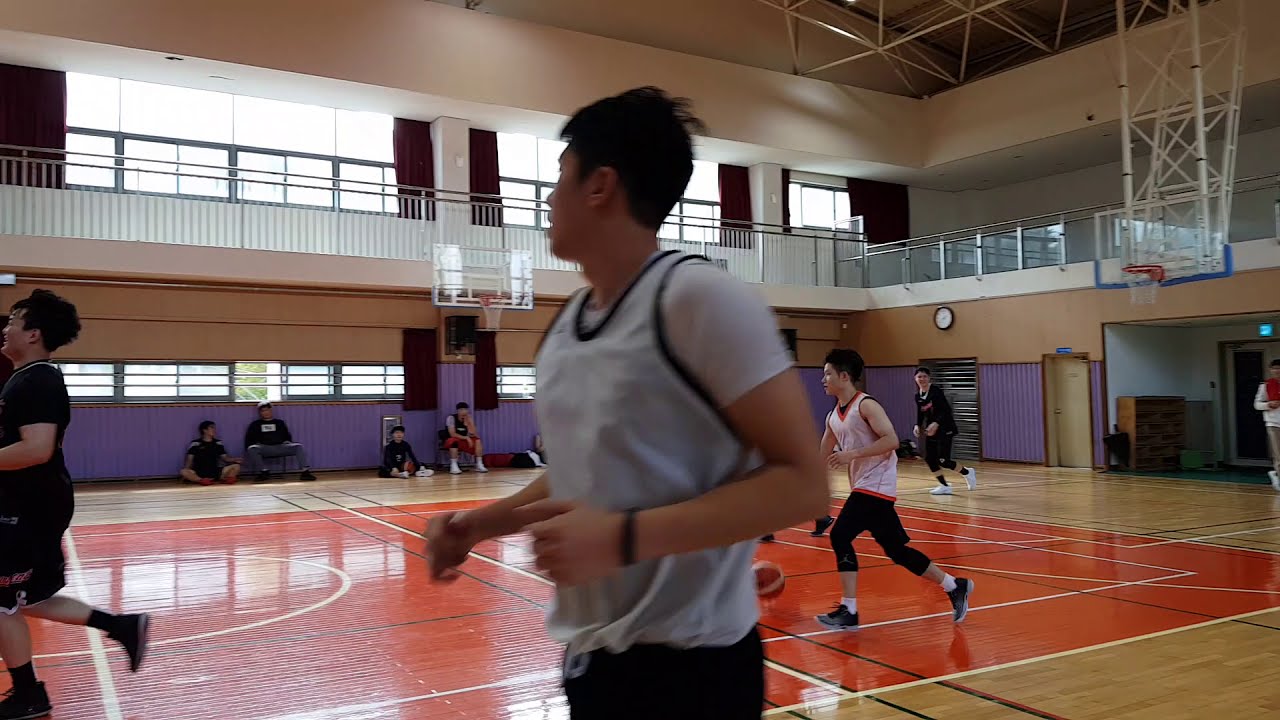The image captures an action-packed moment during an intimate basketball game in a small gymnasium, likely situated in Japan. The gym lacks bleachers but features a balcony with potential spectator space above the court, separated by a glass railing. The basketball hoops, equipped with glass backboards and red rims, hang down from white metal rafters on the ceiling. The court itself is predominantly orange in the center with white lines, bordered by light brown wood tones.

In the foreground, a player with black hair, wearing a white jersey with blue trim and blue shorts, is running down the court, slightly blurred due to the motion. Behind them, another player dribbles the ball, while a third player in a dark-colored jersey, possibly black, sprints alongside, smiling. Several other players are visible, each donning attire that distinguishes their team, including white tops with red piping and black shorts. The lower walls of the gym are purple with tan above, and a few people are seated against the wall, watching the game unfold. The background also hints at a multi-story structure typical of Japanese architecture, with windows offering glimpses of nearby buildings.